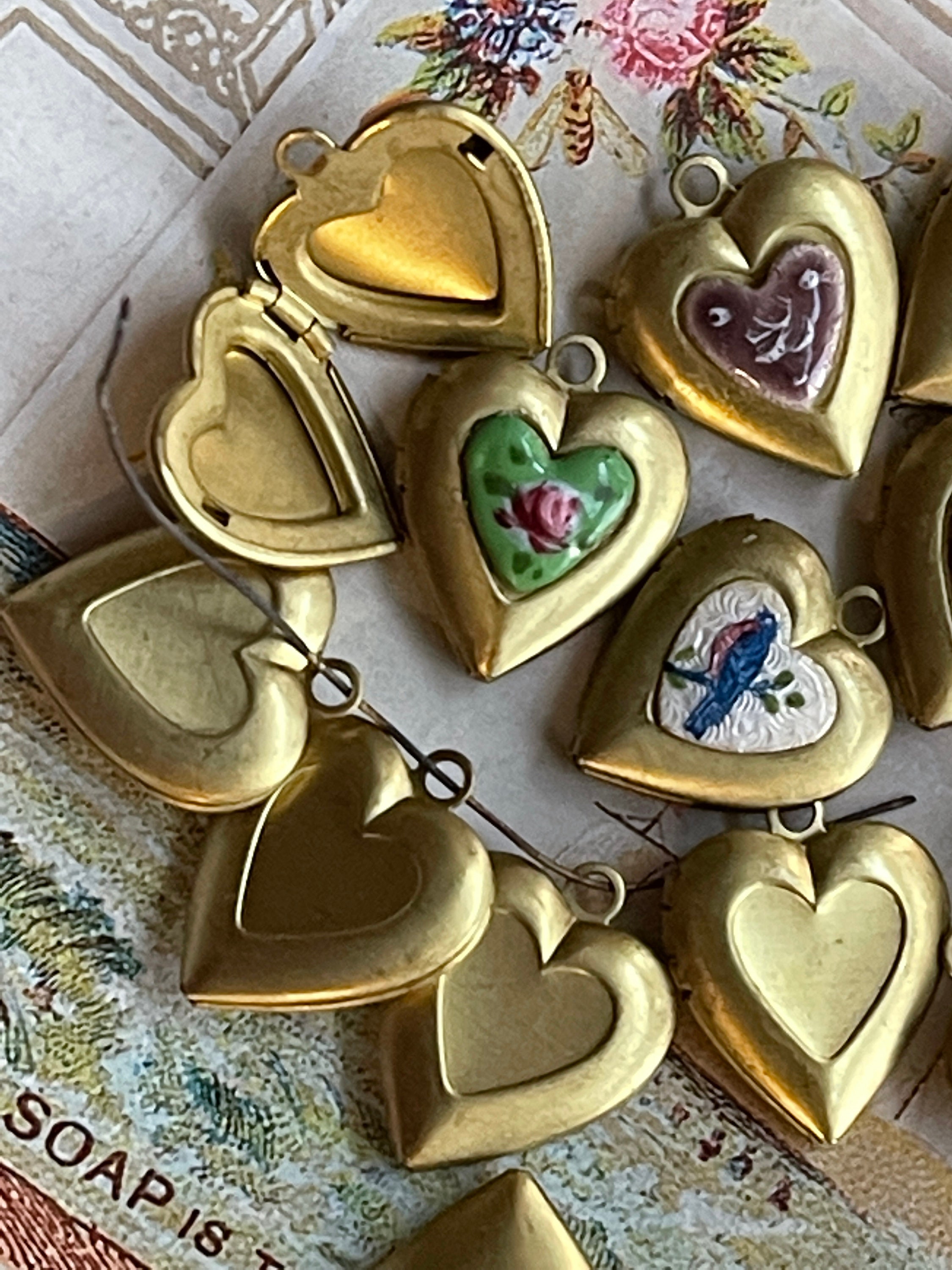This color photograph features a collection of ten small, heart-shaped lockets, primarily gold-colored, resembling brass. These lockets are arranged on a tan item adorned with vintage-style floral patterns, displaying hints of pink and blue flowers. The lockets are distinctly detailed, each with a unique design on the front; some have an indented heart shape, while others boast painted illustrations. Among the illustrated lockets, one presents a red rose on a green background, another depicts a bluebird perched on a branch against a white background, and a third showcases a flower with pink and red hues on green. One of the lockets, positioned at the top left, is open, showing an empty interior. Each locket includes a small gold hoop at the top for threading onto a necklace or similar chain. Additionally, some lockets are aligned in a row on a thin metal wire.